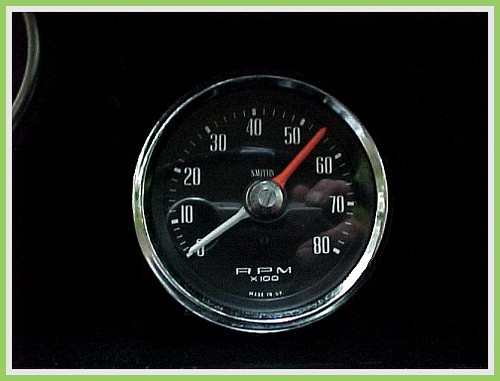This photograph features a close-up view of a car's tachometer, an instrument used to measure the vehicle's engine RPM. The tachometer gauge is round with a chrome rim, providing a sleek and polished look. Set against a black background, both the instrument and the photograph exude a sophisticated ambiance. 

The face of the tachometer itself is black, contrasted by white numbers and lines, which mark the RPM levels. The needle of the gauge, silver in color, is positioned at zero—indicating that the car's engine is not running at the moment. 

A notable feature of the tachometer is the redline area, located between the 5,000 and 6,000 RPM marks, signaling the danger zone for engine performance. Crossing into this red zone would suggest that the engine is revving too high, posing a risk of damage. 

Overall, the image captures every intricate detail of the tachometer, from its sleek chrome border to the critical redline, encapsulated in a dramatic black backdrop.